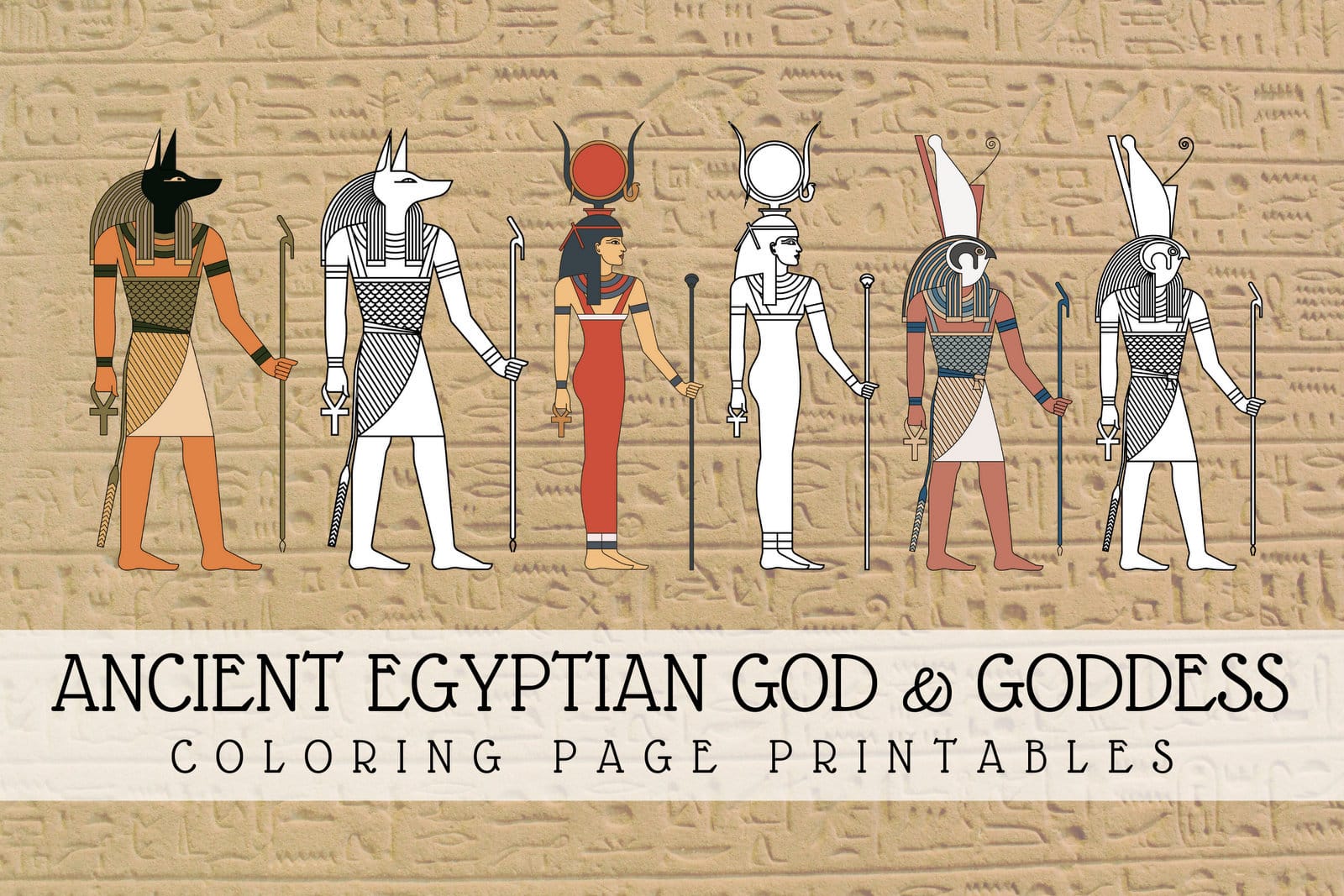This image features a striking banner graphic with a background resembling a beige sandstone wall adorned with detailed rows of ancient Egyptian hieroglyphics, arranged in parallel lines. Across the middle, six cartoonish illustrations of Egyptian deities are displayed. These are divided into pairs, where a fully-colored depiction on the left is mirrored by a black-and-white version on the right, designed as a coloring book page.

The first character on the left is Anubis, illustrated with a black jackal head and a human body, adorned in an orange garment and holding both an ankh and a rod. Directly next to him is his black-and-white counterpart. In the center stands a goddess, likely Isis or Hathor, identified by a large brown sun disc set between two horns on her head, dressed in a form-fitting brown gown with flowing black hair. Her black-and-white equivalent is positioned beside her. The last pair features a figure resembling Toth, depicted with a hawk head and crowned with the double crown of Egypt, also brandishing a rod. This figure, too, has a monochrome version adjacent to it.

Below these illustrations, a prominent gray banner stretches across the bottom, with bold black text declaring "Ancient Egyptian God and Goddess Coloring Page Printables" in an ancient-styled font.